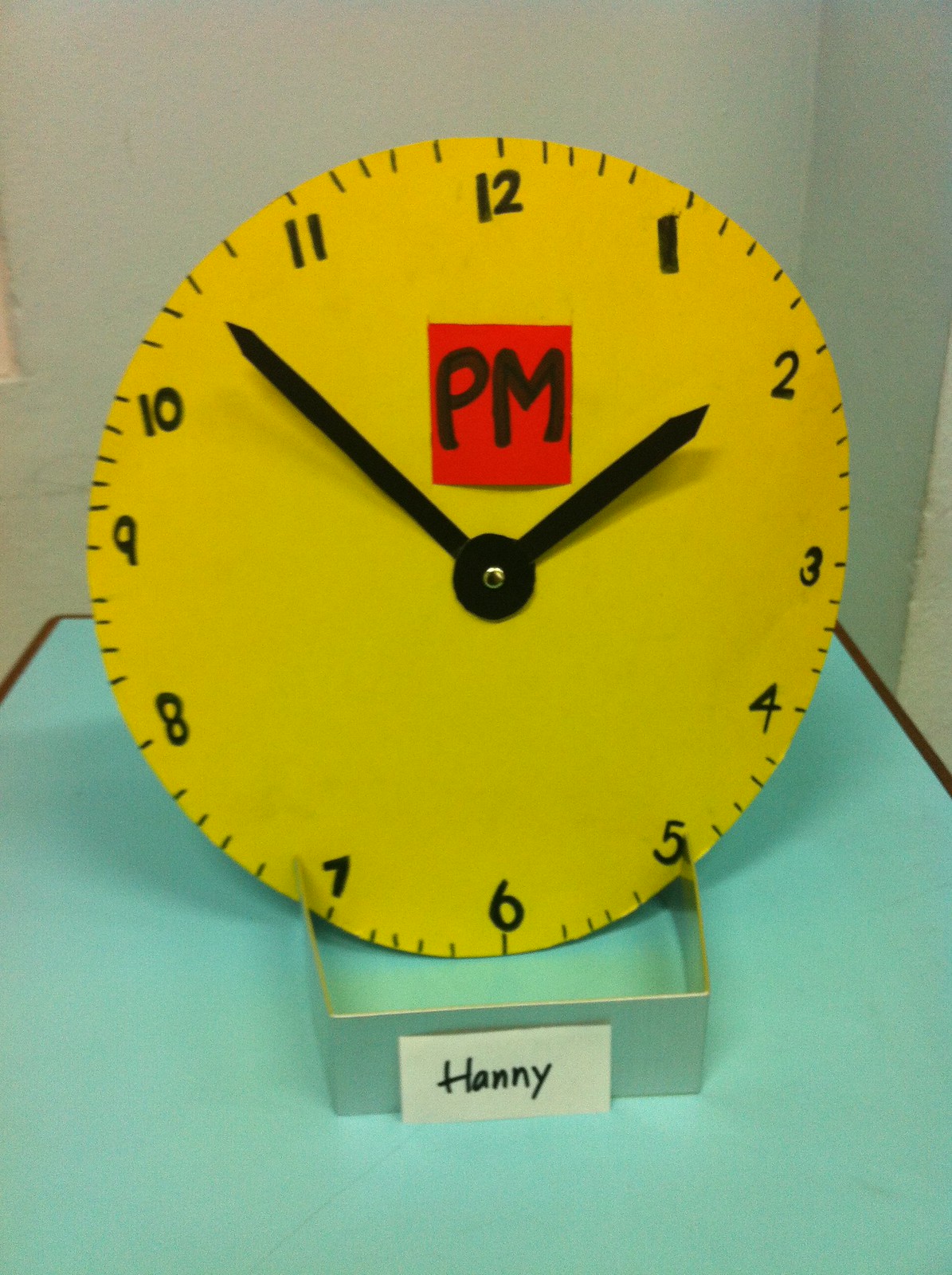This vertically oriented photograph features a homemade clock art project, prominently displayed on a teal rectangular base, which may either be construction paper or the color of the table. The focal point of the image is a large, yellow circular clock. The clock face is meticulously detailed with black marker, indicating both the numbers and the hash marks between numerals, ensuring precise time measurement.

The clock features hour and minute hands, fashioned from black, likely construction paper, adding a tangible, hand-crafted quality to the piece. A red square marked "PM" in black letters is positioned between the center of the clock and the 12, subtly indicating the time period.

At the bottom of the display, a three-sided freestanding object supports a name tag spelling out "HANNY" in bold, black letters. This name tag leans against the object, suggesting that the art project likely belongs to HANNY, possibly created for a school assignment. This vibrant, personalized clock project encapsulates both creativity and educational effort, showcasing HANNY's attention to detail and artistic expression.